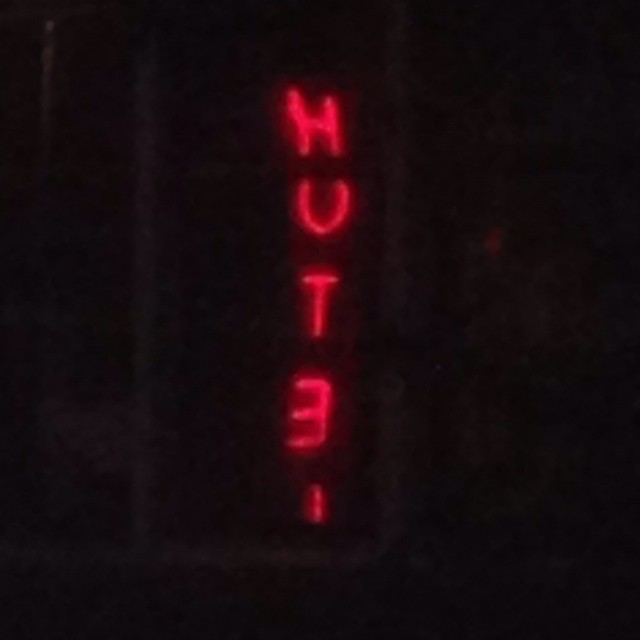This is a color photograph taken at night, featuring a slightly blurry scene with very dim lighting. Dominating the center of the image is a vertical neon or digital display, illuminated in red against a predominantly dark backdrop. The sign displays the letters "H U T E," but the final character is obscured, leaving it partially hidden. The image's background transitions from a dark, almost black shade on the left and right sides to a slightly lighter gray on the top left corner, delineated by faint vertical pillars and horizontal lines. The overall ambiance is mysterious and unclear, adding intrigue to the setting of the sign.